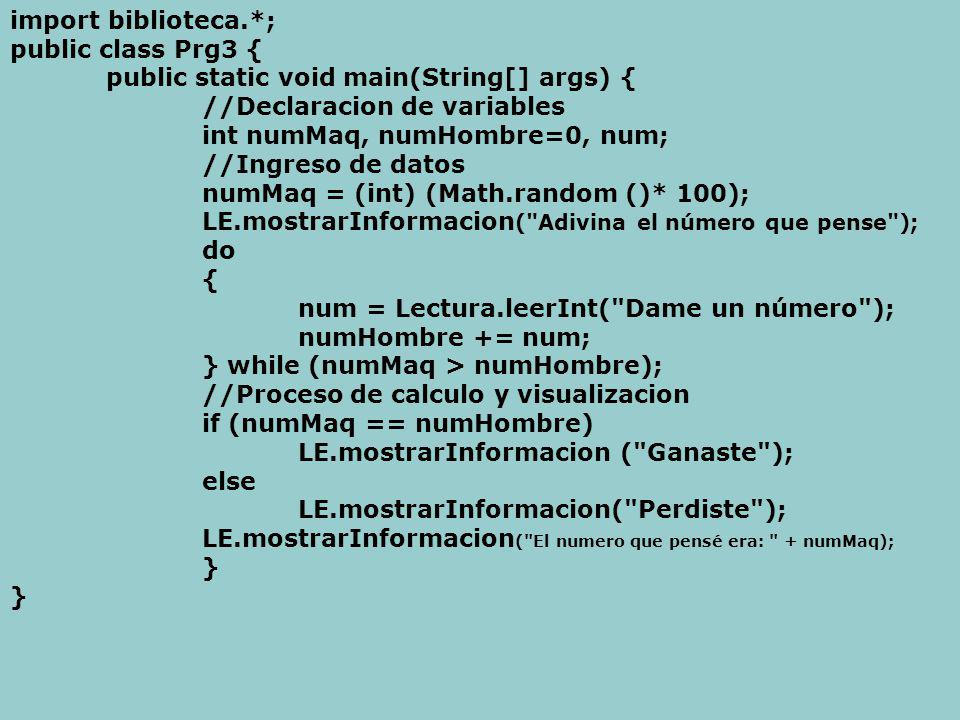The image depicts a detailed snippet of computer code, displayed against a light blue background with bold black text. The code includes both English and Spanish elements. At the top left corner, it begins with 'Import Bibliotheca Fabiostar;' followed by 'public class PRG3'. The code structure is clearly formatted with curly brackets enclosing several indented sections. Key elements include 'public static void main(String[] args)', and Spanish declarations such as 'declaration de variables' and 'int numMack numUmbrae = 0'. The code continues with variable declarations, input prompts ('numIngresoDeDatos'), and control structures including 'if statements'. The centralized section features mathematical operations ('Math.random(100)', 'lay.mostrarInformacion(adivinaElNumeroQuePensado)'). The syntax seems oriented in a left-justified manner, with some sections more centered. The detailed Spanish lines indicate processes like 'numLectura.layerIntDeUnNumero' and logic handling for winning scenarios ('le.mostrarInformacion(ganaste)'). Overall, it is a comprehensive piece of programming code, meticulously blending English and Spanish terminologies to manage a numerical guessing game algorithm.